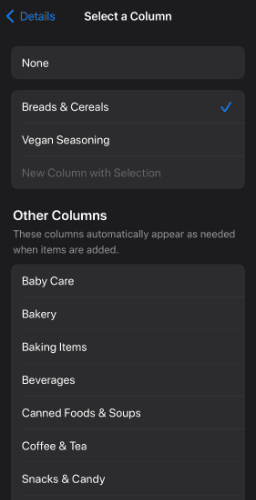This image, captured from a cell phone screen, showcases a predominantly black background. At the very top left-hand corner, there's a blue arrow icon followed by the word “Details” in blue, indicating a link or button. The main header below reads “Select a column,” with all text in this section appearing in white. Each text element is positioned within nearly black, slightly grayish rectangles, giving a subtle contrast to the background.

Below the header, the first option listed is “None.” Further down, within this structured format, the section labeled "Breads and Cereals" is highlighted by a blue checkmark next to it. This is the only checkmark on the page. Underneath, it indicates "Vegan Seasoning" and an option to "New column with selection," suggesting the ability to add more categories.

Continuing down, there’s a subheading labeled "Other columns," explaining that "These columns automatically appear as needed when items are added." Following this, a list of items appears in white text: "Baby Care," "Bakery," "Baking Items," "Beverages," "Canned Foods and Soups," "Coffee and Tea," and "Snacks and Candy." The visual layout and color scheme emphasize a clear, organized interface for easier navigation and accessibility.